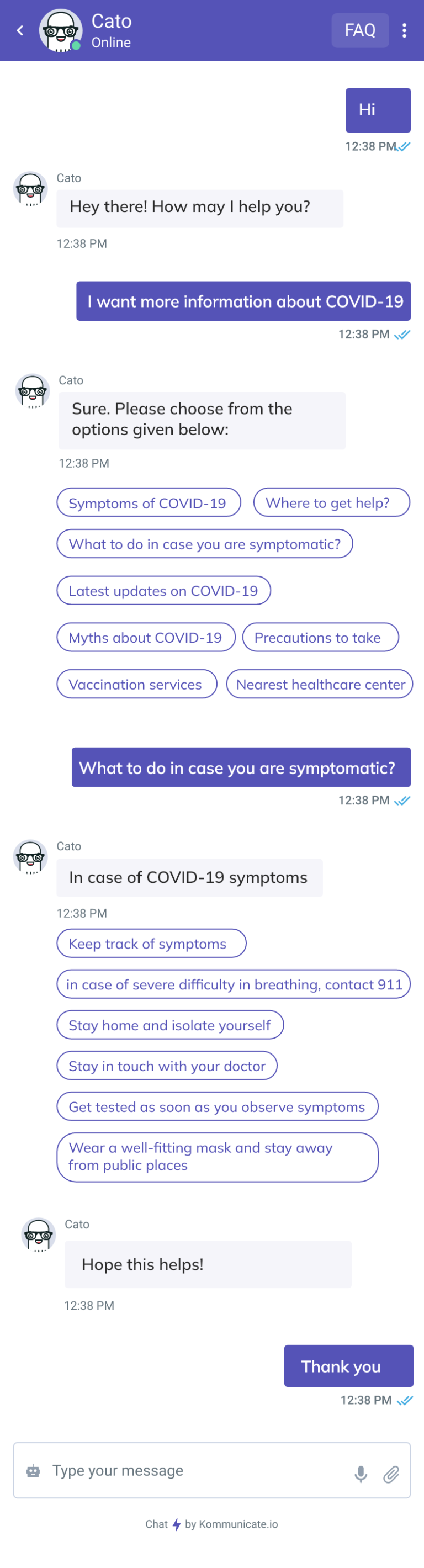The image is a screenshot featuring a digital FAQ interface for Cato, with a white background. At the top, there are the words "Cato FAQ" along with three vertical dots, typically indicating a menu or additional options. The interface comprises both purple and gray rectangles.

The upper section includes two main rectangles: a purple one containing a chatbot greeting, saying, "Hey there, how may I help you?" followed by a user’s response in a gray rectangle, "I would like more information about COVID-19."

The chatbot replies affirmatively in another purple rectangle, providing a range of clickable options for detailed information. These options include:
- Symptoms of COVID-19
- Where to get help
- What to do in case you are symptomatic
- Latest updates on COVID-19
- Myths about COVID-19
- Precautions to take
- Vaccination services
- Nearest health care center

Following this, there is an expanded section on "What to do in case you are symptomatic," highlighted with a purple header. Beneath this, a gray rectangle outlines specific steps, such as "Keep track of symptoms," and continues with a list of instructions.

The interface concludes with a message in a purple rectangle saying, "Hope this helps," followed by a user’s response, "Thank you," and at the very bottom, a text input field with the prompt "Type your message." Adjacent to this field are small icons for a camera on the left, and a microphone and paperclip on the right, suggesting options for multimedia inputs or attachments.